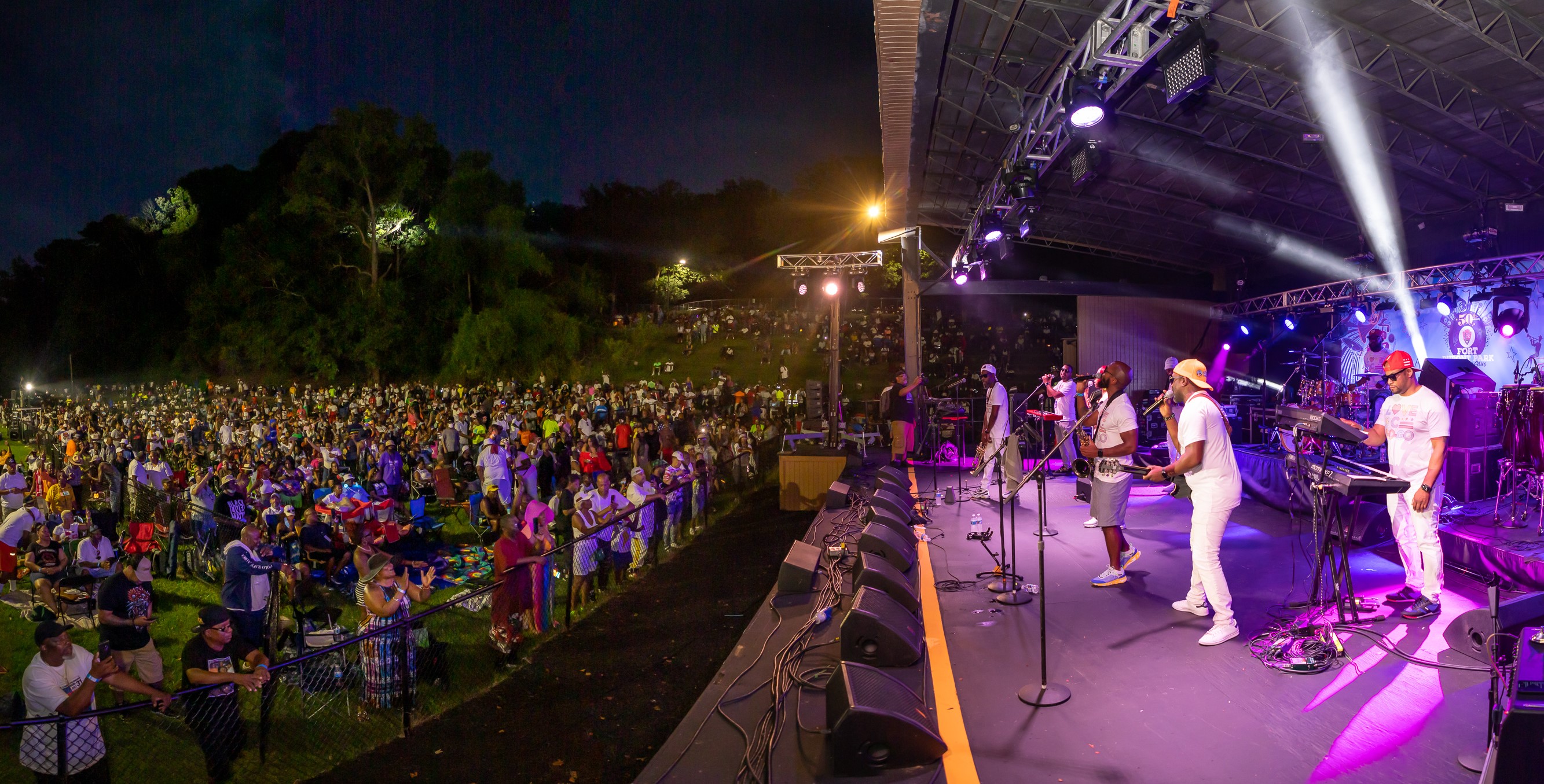The image captures a vibrant nighttime concert set on a green field, with big trees in the background. The crowd, which completely fills the field, is separated from the stage by a black chain-link fence. The stage itself is framed with gray steel girders and has an overhang. It's illuminated with beams of purple and blue light emanating from various spotlights and flashlights. At the front of the stage, there are multiple black speakers, a variety of wires, and mic stands. The performers on stage, comprising a band of black musicians, are all wearing white t-shirts. You can see them engaged in their performance with two guitarists, a keyboard player positioned near the front, several singers at microphones, and a drum set in the background. The audience is a mix of people leaning on the fence, standing, and sitting, all engrossed in the show. The entire scene embodies the lively atmosphere of a nighttime outdoor concert.